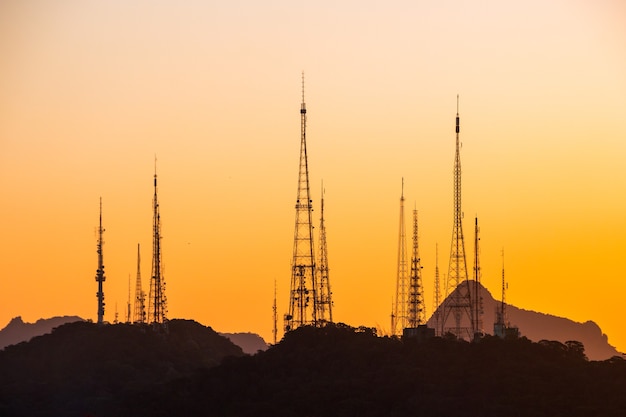The photographed image features a striking display of numerous radio towers, ranging between 14 to 20 in number, extending vertically against a predominantly golden-orange sky. The color gradient shifts from a deep, dark gold near the base to a light, pastel hue at the top. The towers, silhouetted in black, have a metal grid structure forming tall and narrow pyramid shapes with wide bases tapering to pointed tips. This scene appears to be captured either at dawn or dusk, as suggested by the golden hue of the sky indicating the sun is just below the horizon. At the base of these towers, a series of hills or mountain ranges spans across the lower 20% of the image, blending into dark outlines with some vegetation visible. Among the hills in the foreground, which are distinctly black, some buildings can be seen overshadowed by the towering structures, which rise at least 100 feet above them. The hills in the background appear hazy and are a lighter dark, almost sepia-toned. The tallest tower stands prominently a little left of center, with the next tallest positioned towards the middle of the right half of the image, and the rest varying in height and distance, adding depth to this captivating landscape.